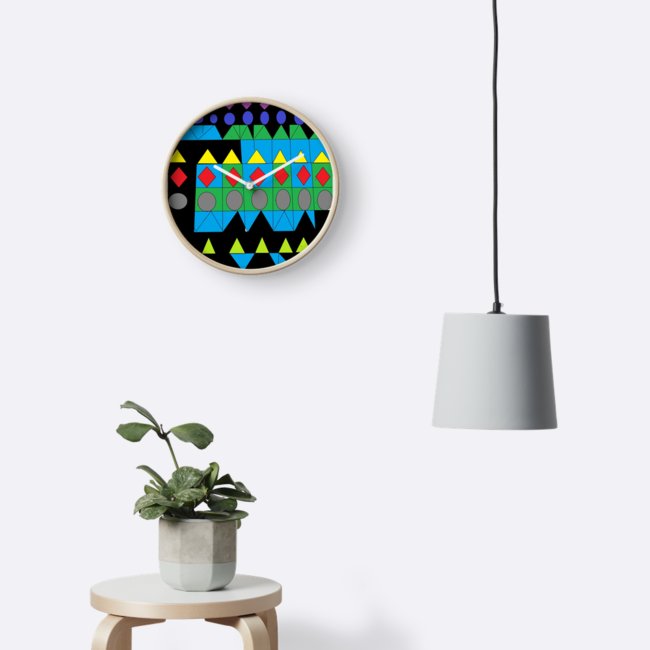The image captures a minimalist, yet vibrant interior scene with a striking white wall backdrop. Dominating the lower left corner is a tan wooden stool featuring three legs, upon which rests a distinctive gray, rounded flower pot divided into three sections, housing a small green plant. Above it, a whimsical round clock hangs slightly left of center on the wall, displaying the time at approximately 10:10. The clock face is adorned with a colorful, geometric pattern comprising gray circles, red diamonds, yellow triangles, blue triangles, and green triangles, set against a black background with white hands but no numbers. To the right, about halfway down the photo, a lamp fixture descends from the ceiling via a long black cord, leading to a white lampshade that tapers slightly towards its base, casting light onto the scene. The simplicity of the setup, combined with the playful decor elements, gives it a chic, contemporary vibe reminiscent of stylish online home decor displays. A subtle shadow is cast by the plant and stool, adding depth to the composition.